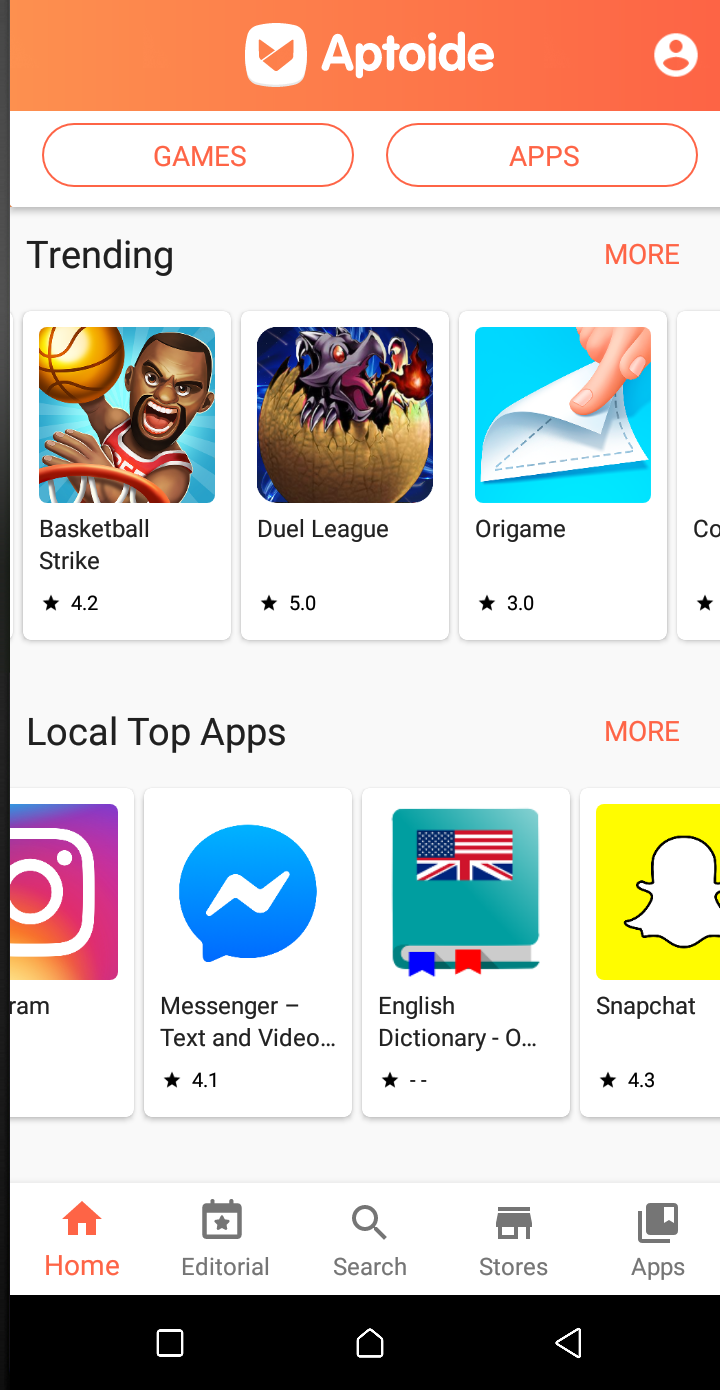**Detailed Caption:**

The image appears to be a screenshot of a mobile phone displaying the main interface of the Aptoide app store. 

At the very top of the screen is an orange bar. Within this bar, slightly to the left, there is a white square followed by an orange triangle pointing downward, resembling an incomplete "play" button. To the right of these symbols, the word "Aptoide" is written in white capital letters.

Below the top bar, there is an icon of a little orange head and shoulders within a circular border.

Underneath this, a large white rectangular section contains two prominently outlined buttons with rounded corners and orange borders. The first button is labeled "Games" in orange letters, and the second button is labeled "Apps," also in orange letters.

Following this, there is a horizontal gray bar with the text "Trending" in black lettering on the left and "More" in orange lettering on the right.

Further down, within a larger white square, there are multiple smaller rectangular boxes, each representing different app icons with titles and descriptions. 

1. The first box features a game called "Basketball Strike," illustrated with an image of a basketball hoop and a black cartoon character dunking a basketball.
2. The second box titled "Duel League" shows an image of Earth with an alien emerging from it.
3. The third box is labeled "Origami" and it displays a person's finger folding a piece of paper.

Below these app icons, a section header titled "Local Top Apps" is written in black letters on the left, with the word "More" in orange letters on the right.

The subsequent section displays several popular apps, each within their own white rectangle:
- "Instagram," paired with its recognizable multi-colored camera icon.
- "Messenger," denoted by a blue speech bubble icon.
- "Video" and "Inside," also represented within the same visual context as Messenger.
- "English Dictionary," symbolized by a green icon featuring a British flag and a blue and red bookmark within the green book imagery.
- "Snapchat," marked by its iconic yellow square containing a white ghost.

At the very bottom of the screen, there is another white rectangular section with icons for "Home," "Editorial," "Search," "Stores," and "Apps," suggesting navigation tabs for different sections of the Aptoide app.

Finally, a black bar at the bottom of the image features three icons in white: a small square, a house, and a left-pointing triangle, which likely represent additional navigation buttons for the device.

This detailed description encompasses all the elements visible within the screenshot, giving a clear and thorough breakdown of the visual information displayed.